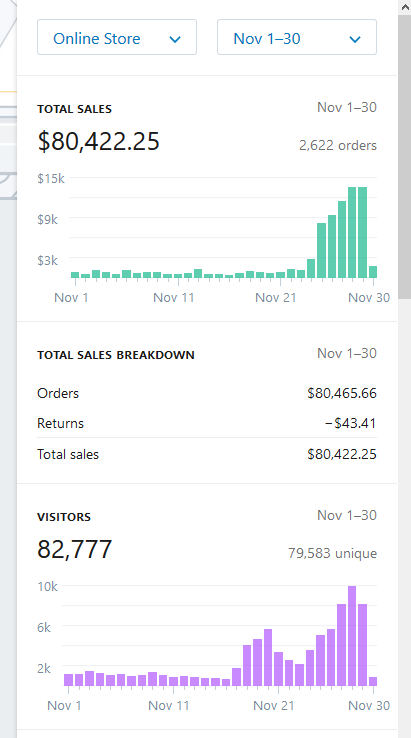Screenshot Caption: 

A detailed performance dashboard for an online store, displaying sales data for the period of November 1-30. The dashboard has a white background and prominently features key metrics in blue. 

Key statistics include:
- Total Sales: $80,422.25, generated from 2,622 orders.
- Visitors: 82,777 in total, with 79,583 being unique visitors.

A sales chart plots total sales over the month, marked on dates Nov 1, Nov 11, Nov 21, and Nov 30 against Y-axis markers of 3k, 9k, and 15k sales. Notable points on the chart show:
- Approximately $1.4k on Nov 1
- Around $1.1k on Nov 11
- About $1.4k on Nov 21
- Peaking roughly at $13k on Nov 30

Additionally, a breakdown of total sales from Nov 1-30 includes:
- Orders amounting to $80,465.66
- Returns valued at -$43.41
- Resulting in net total sales of $80,422.25